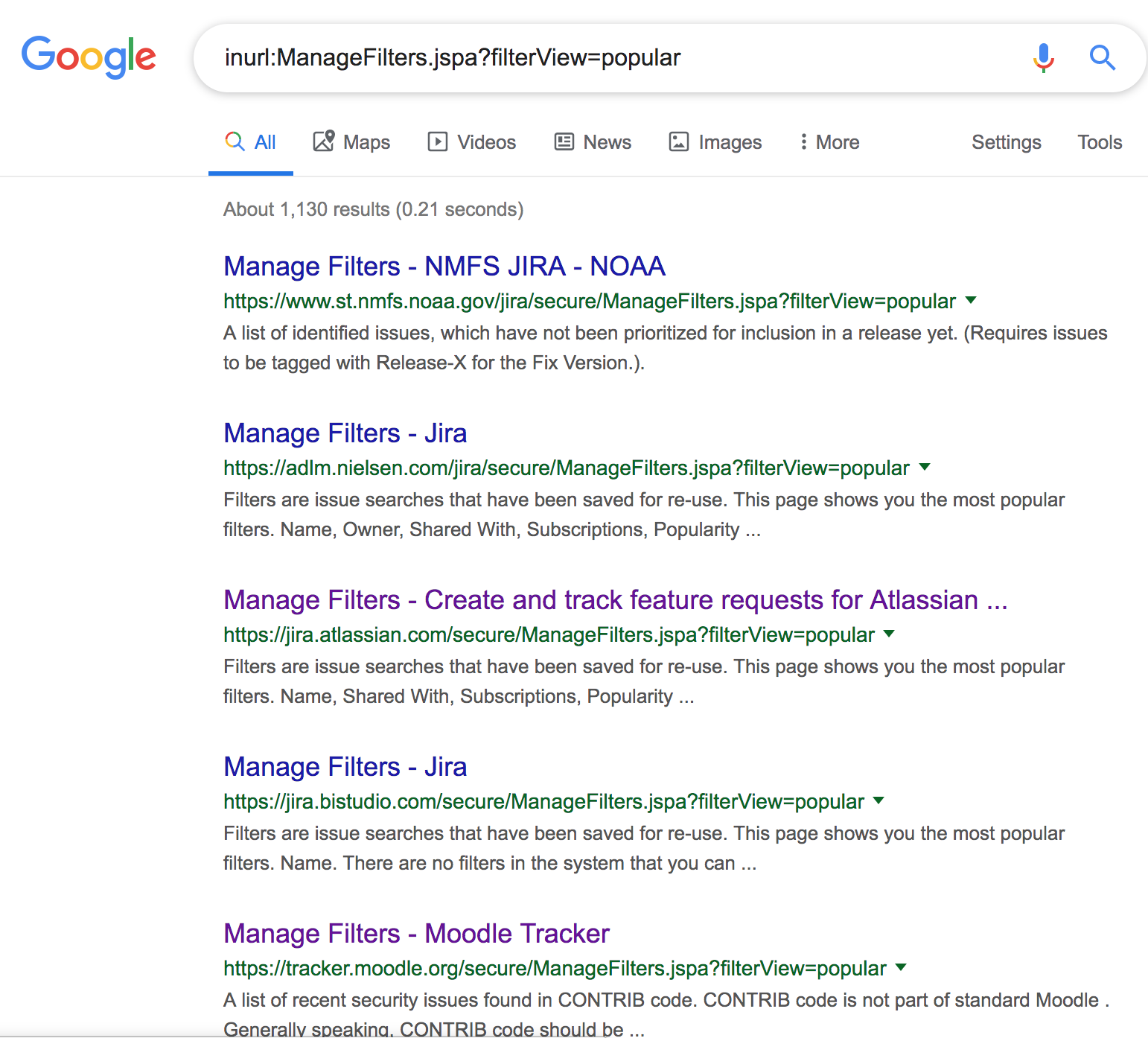The image displays a Google search results page. The background is predominantly white. In the top left corner is the iconic Google logo, rendered in its trademark colors of blue, red, yellow, and green. Below the logo lies an oval-shaped search box containing the search query "inurl.managefilters.jspa?filterview?popular" displayed in black text.

Directly beneath the search box, there is a navigation menu with clickable options. The first option, "All," is highlighted in blue, indicating it is currently selected. Other menu options next to it include "Maps," "Videos," "News," "Images," "More," "Settings," and "Tools."

Below this navigational bar is a thin gray line that spans the width of the page. Underneath this line, the text reads "About 1,130 results (0.21 seconds)," indicating the number of search results and the speed of the search.

The search results are listed as follows:
1. **Managefiltersnmfsjira-noaa** (first choice)
2. **Managefilters-jira** (second choice)
3. **Managefilters create and track future requests for Atlassian** (third choice)
4. **Managefilters-jira**
5. **Managefilters-moodletrack**

The links to these results are in blue text, except for the third result, which has been clicked on previously and turned purple, signifying it has been visited before. This illustrates the behavior that links change color when clicked.